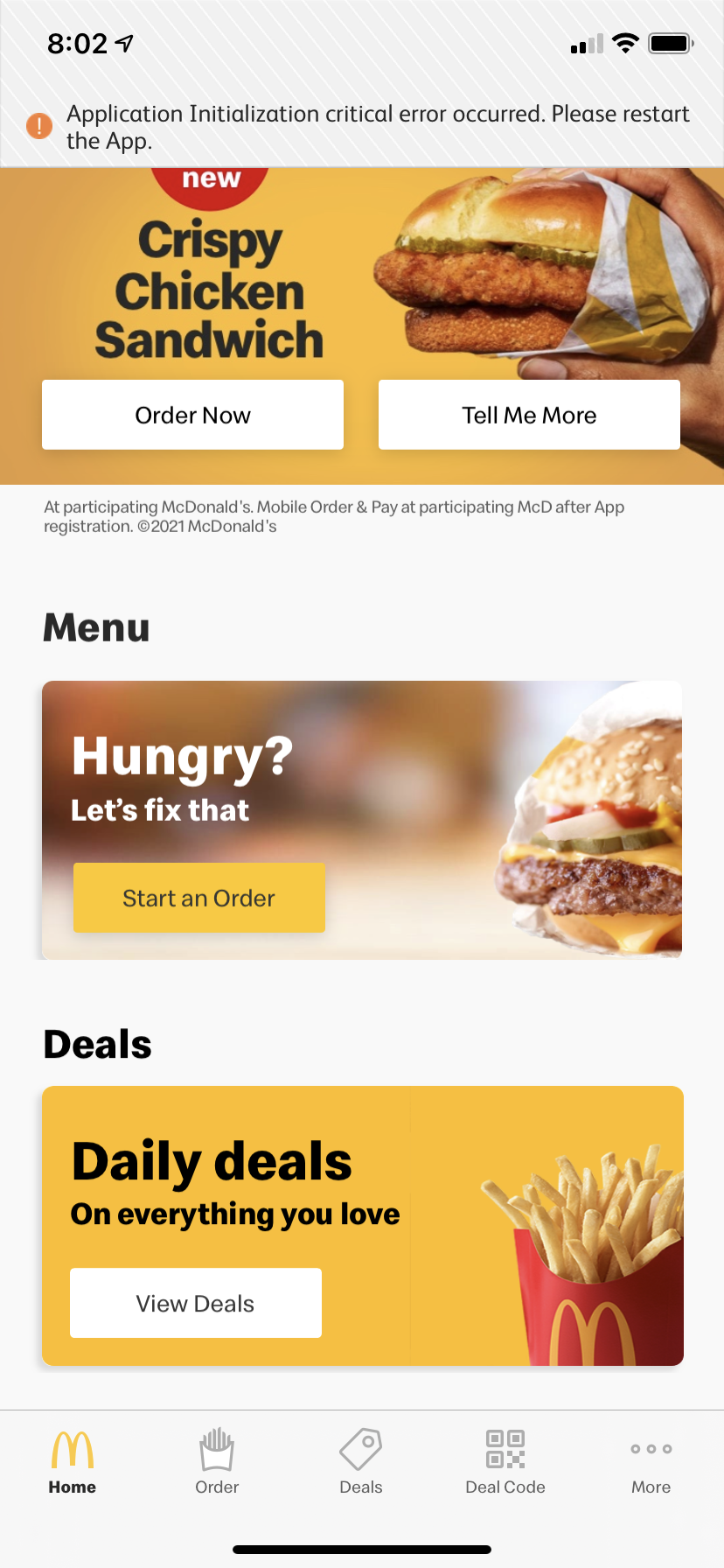A detailed screenshot of the McDonald's mobile app interface is depicted. At the top of the screen, within the status bar containing the time and signal indicators, there is a prominent alert reading, "Application Internalization Error. Critical error occurred. Please restart the app." Below this alert, the app's main promotional section can be seen, featuring an advertisement for McDonald's crispy chicken sandwich. The ad includes an image of a hand holding the crispy chicken sandwich along with clickable buttons labeled "Order Now" and "Tell Me More." In smaller text beneath the ad, information about participating McDonald's locations for mobile orders and required app registrations is displayed.

The color scheme of the app predominantly comprises white with striking accents of yellow and red that complement McDonald's branding. Following the promotional section, a menu banner is visible, accompanied by a tagline that reads, "Hungry? Let's fix that. Start an order." Adjacent to this tagline there is a detailed image of a premium burger, suggesting it's not a Big Mac but a higher-tier menu item.

Further down the screen, there is another banner advertising deals with the text, "Daily deals on everything you love." A "View Deals" button is prominently placed within this section, and the image alongside it shows a close-up of McDonald's iconic french fries in the characteristic red holder with the yellow 'M' arch logo.

At the very bottom of the screenshot, the app's navigation bar is visible, offering shortcuts labeled "Home," "Order," "Deals," "Deal Code," and "More."